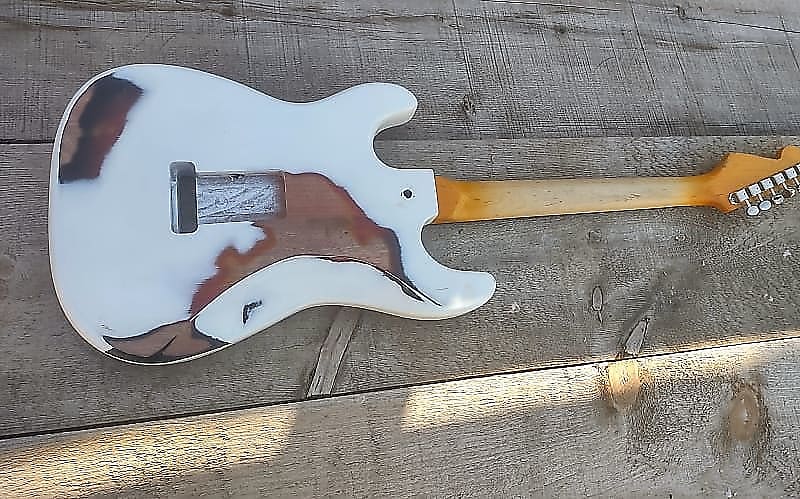The image showcases a distressed white electric guitar with a high-quality wooden fretboard, devoid of strings, lying horizontally on a weathered wooden surface. The body of the guitar exhibits brown abstract patches, contributing to its unique and worn design. The setting, likely an outdoor porch, features a grey, grainy, and chipped wooden floor, enhancing the rustic aesthetic. Light filters through, suggesting the photo was taken during the day in a shadowed area. The guitar's construction appears to be a mix of wood and possibly plastic, with the round base positioned to the left and the fret to the right. The back of the guitar displays a hollowed rectangular area, hinting that it might also be nailed to a wall.